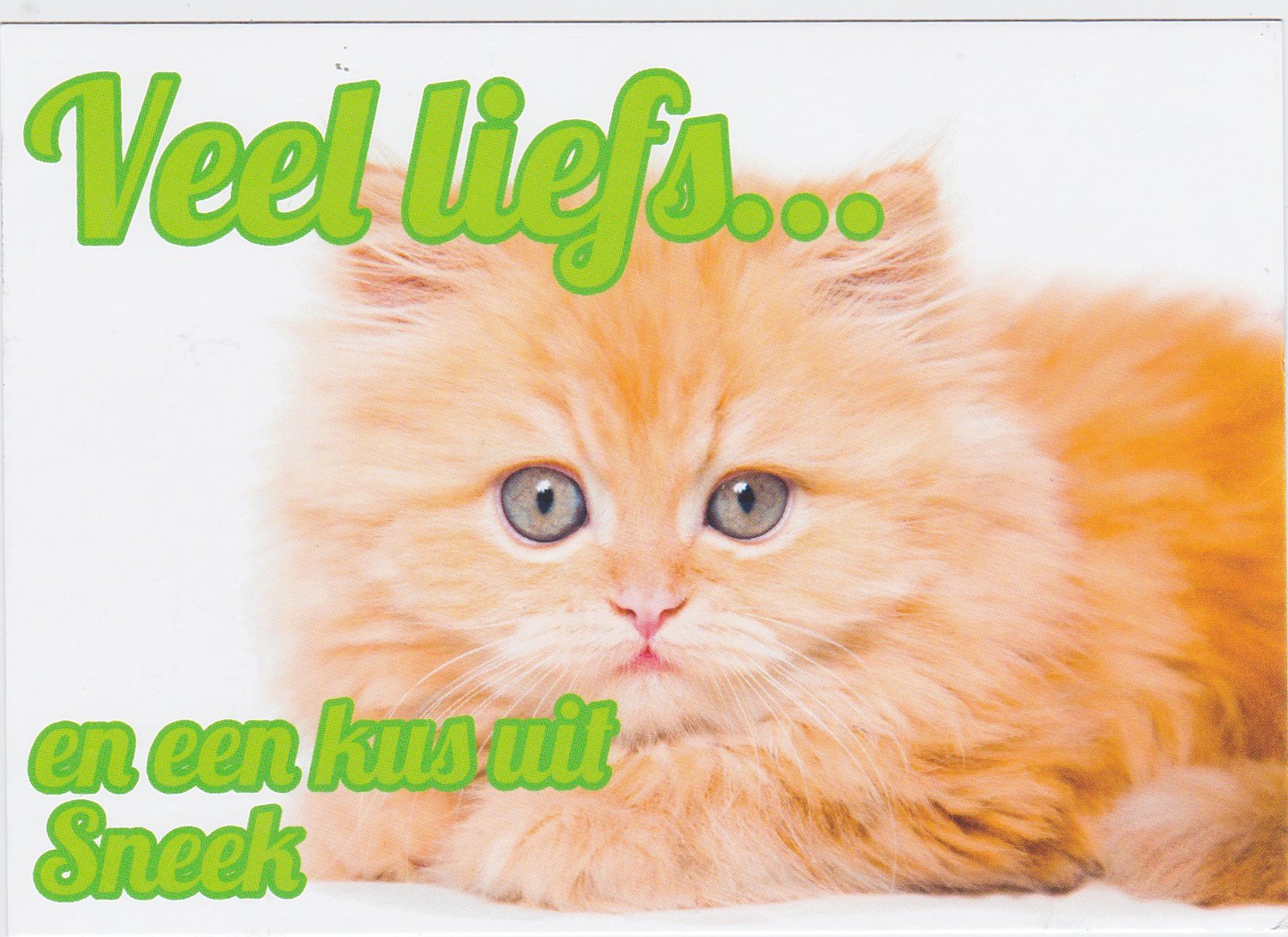In this photograph, an adorable kitten with light orange fur and slightly darker, more vibrant orange markings towards the back of its small body is seen lying down against a plain white background. The kitten's solemn yet focused expression stands out, with its big, grayish-hazel eyes capturing the viewer's attention. Its pink nose and mouth, complemented by white whiskers, add charm to its face. The kitten's paws are delicately placed in front, supporting its posture as it gazes intently at the camera. At the top of the image, there's a line of text in green letters, intriguingly written as "Veal Lief’s…" and, towards the bottom left, "En In Kooz Uit Sneak," suggesting that the text is in a foreign language and might indicate that the image is part of an internet meme. The scene, presumed to be indoors due to the lack of shadows and sunlight, is simple, featuring just the kitten and the text, creating a minimalist yet captivating composition.